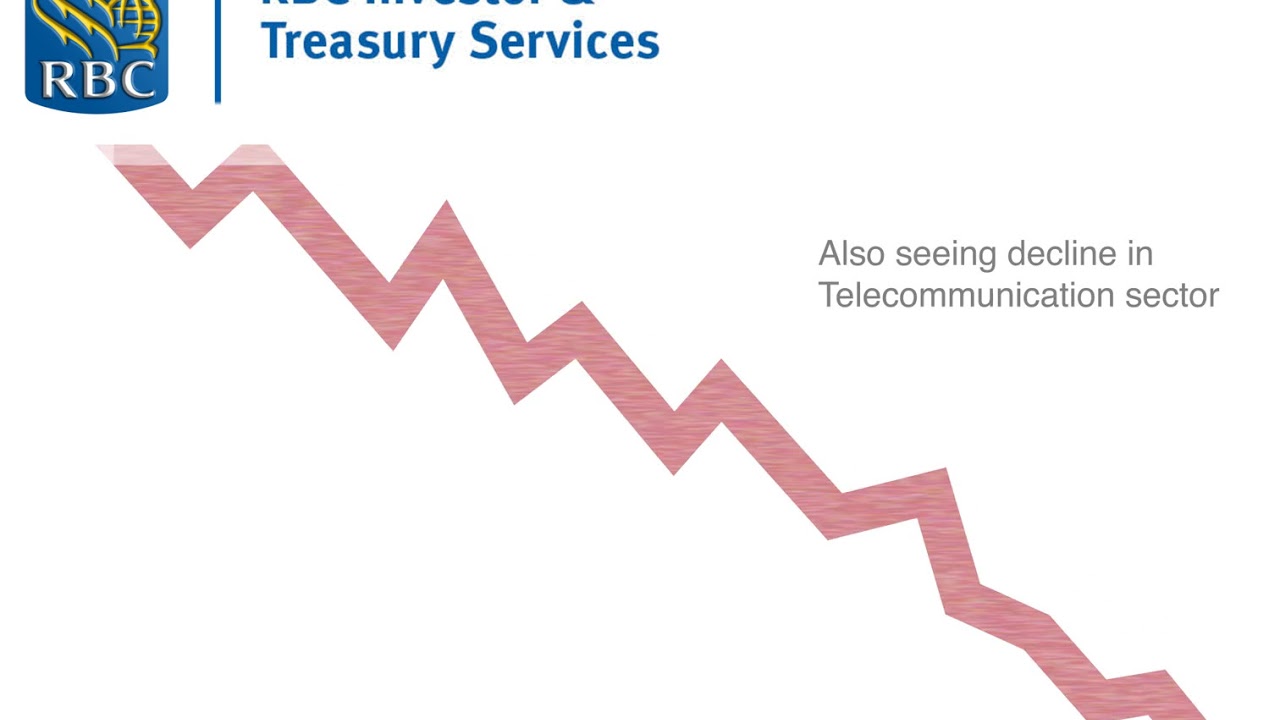The image features a line graph set against a white background, dominated by a light red, zigzagging line that trends downward from the upper left to the lower right. In the top left corner, there is a partially visible blue square logo with yellow designs resembling a globe and leafy patterns, accompanied by the white text "RBC." To the right of the logo, the words "Treasury Services" are clearly visible in blue. The graph itself shows a series of up-and-down movements, predominantly descending, and culminates at a low point on the right side. Central to the graph, there is gray text stating, "also seeing decline in telecommunications sector," indicating that the data likely pertains to financial trends within that industry.